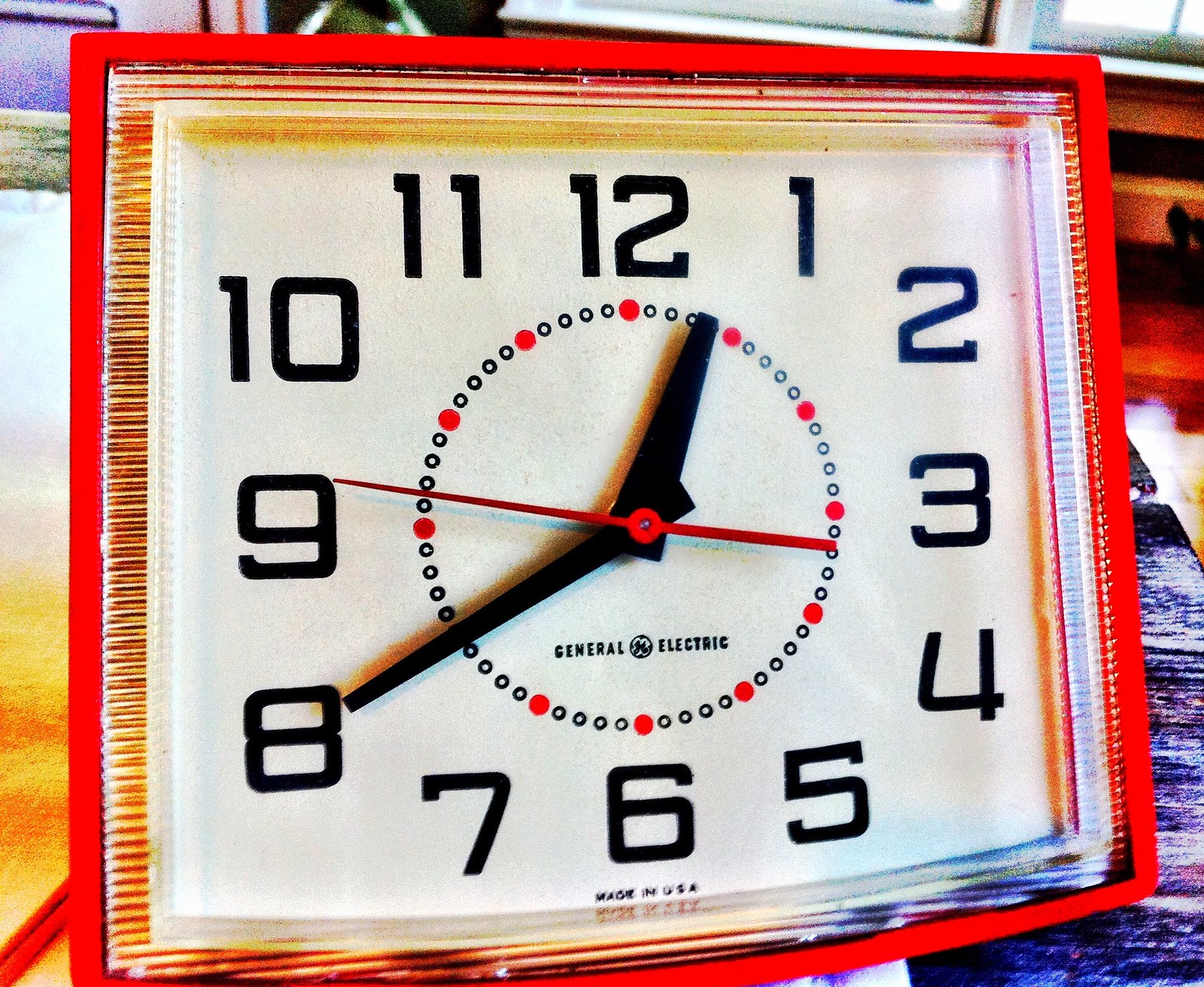This vibrant and detailed color photograph focuses on a square clock, capturing its intricate elements with precision. The clock's frame features a striking red edge, encasing a glass rim adorned with horizontal imprints. The pristine white face of the clock is marked with bold black numerals from 1 to 12, each encompassed by a fully colored red circle, adding a pop of color to the design. Encircling the numerals is an inner ring of petite black dots, providing additional detail.

The clock's time is indicated by two black hands: the minute hand pointing to the 8, and the hour hand situated between 12 and 1. A slender red second hand is positioned slightly past the 9, adding dynamic movement to the image. Below the hands, a black logo reads "General Electric," flanked by a circular emblem. Near the bottom, the text "106 Made in" is visible, though the country of origin is blurred and indiscernible.

In the background, a palette of colors ranging from yellow to blue can be seen on either side, suggesting a lively environment. The clock appears to rest on a bluish surface, while the upper right-hand corner reveals the edge of a window, hinting at a broader setting. This carefully composed photograph not only highlights the clock's design but also situates it within a colorful and engaging context.